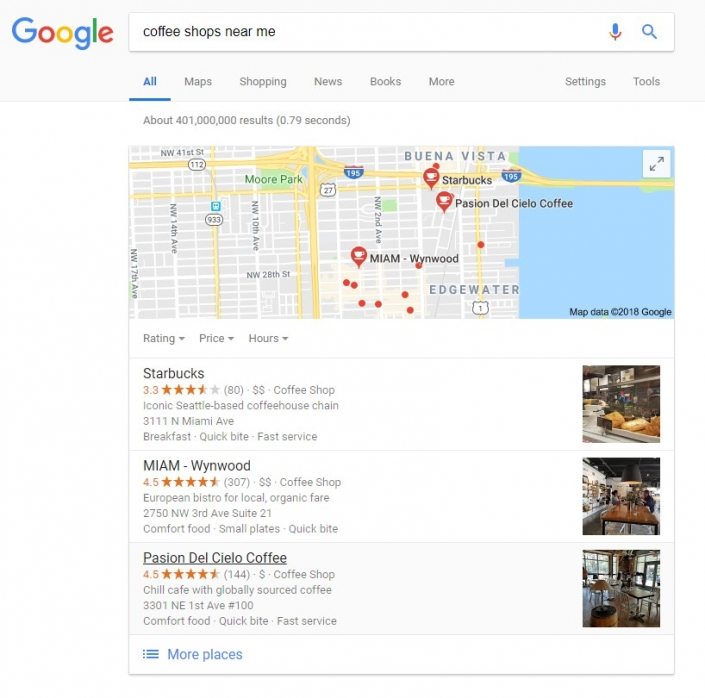The image displays a Google search results page on a website. In the upper left-hand corner, the distinctive Google logo appears in its trademark colors of blue, red, yellow, and green. The search query "coffee shops near me" is prominently highlighted in blue with an underline, indicating it's an active query.

A detailed map is featured, pinpointing various coffee shop locations along what appears to be Buena Vista, likely in Florida. The map is dotted with small red markers denoting the coffee shop locations, accompanied by details such as ratings, price ranges, and hours of operation.

The first listing is for Starbucks, showing a rating of 3.3 stars. The address is listed alongside descriptors like "breakfast," "quick bite," and "fast service." A photograph of the interior of Starbucks is included.

The second listing is Miami Windward, rated at 4.5 stars. It provides the address and tags including "comfort food," "small plates," and "quick bite."

The third and final visible listing is Passchendaele Cielo Coffee, also with a 4.5-star rating. It offers "comfort food," "quick bite," and "fast service," and features a photograph of the shop's interior.

Below these entries, a link marked "More places" appears in blue, suggesting additional coffee shop options are available.